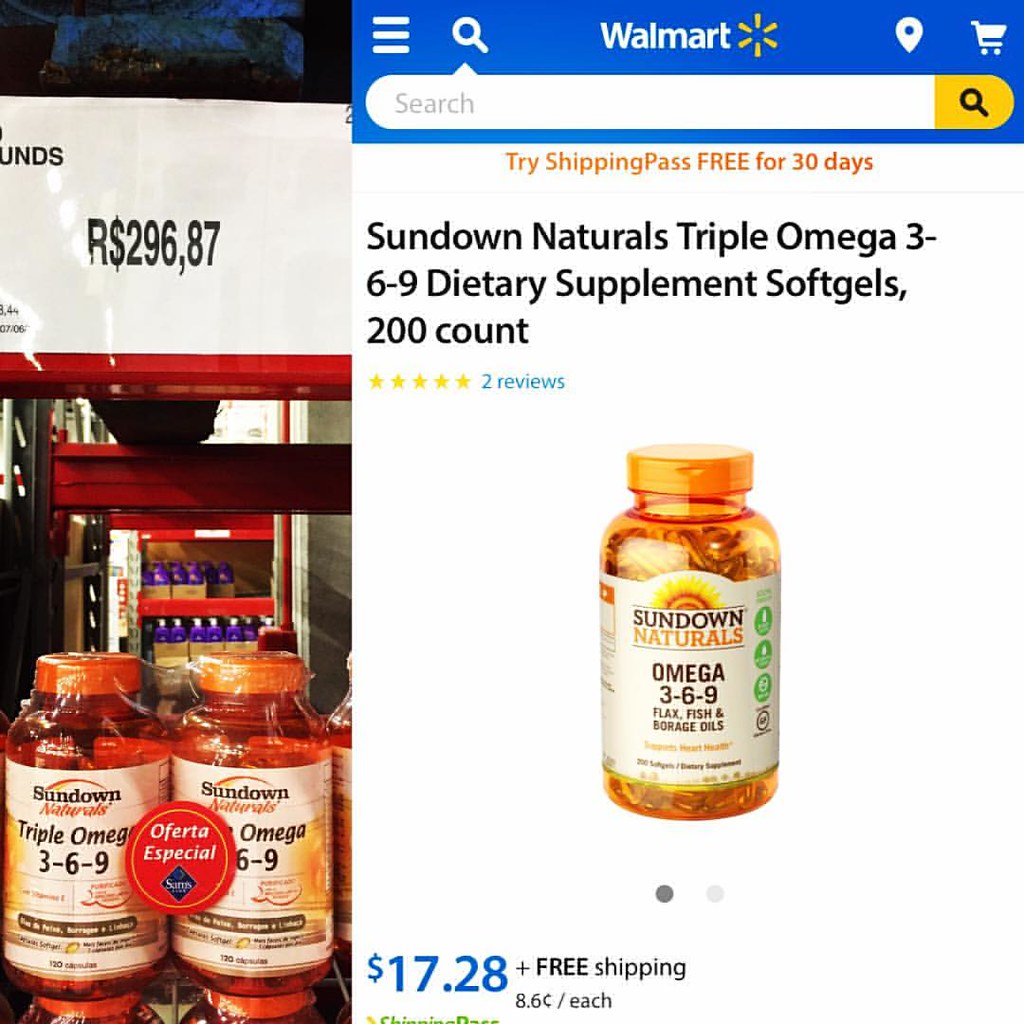The advertisement featured on the Walmart website showcases the "Sundown Naturals Triple Omega 3-6-9" dietary supplement soft gels, presented in a clear orange bottle containing 200 capsules. The bottle's front label prominently displays the brand "Sundown Naturals" and the product name "Omega 3-6-9," highlighting that it includes flax and fish sources. The packaging is adorned with blue-green circles.

The webpage includes a search bar with the keyword "Walmart," indicating the store's branding at the top. The product title "Sundown Naturals Triple Omega 3-6-9 Dietary Supplement Soft Gels, 200 Count" is prominently featured on the page, along with an average rating indicated by stars and the number "2" referencing the available reviews.

The price listed for the product is $17.28, with a note that each capsule costs 8.6 cents, and the product includes free shipping. Further down, there is information about different purchasing options, including an invitation to try the ShippingPass free for 30 days. A side image within the advertisement depicts multiple jars of the supplements, wrapped in plastic and displayed on shelves in what appears to be a warehouse.

Overall, the ad is detailed and informative, providing clear pricing, product count, and highlights a promotion for free shipping, designed to attract potential buyers.